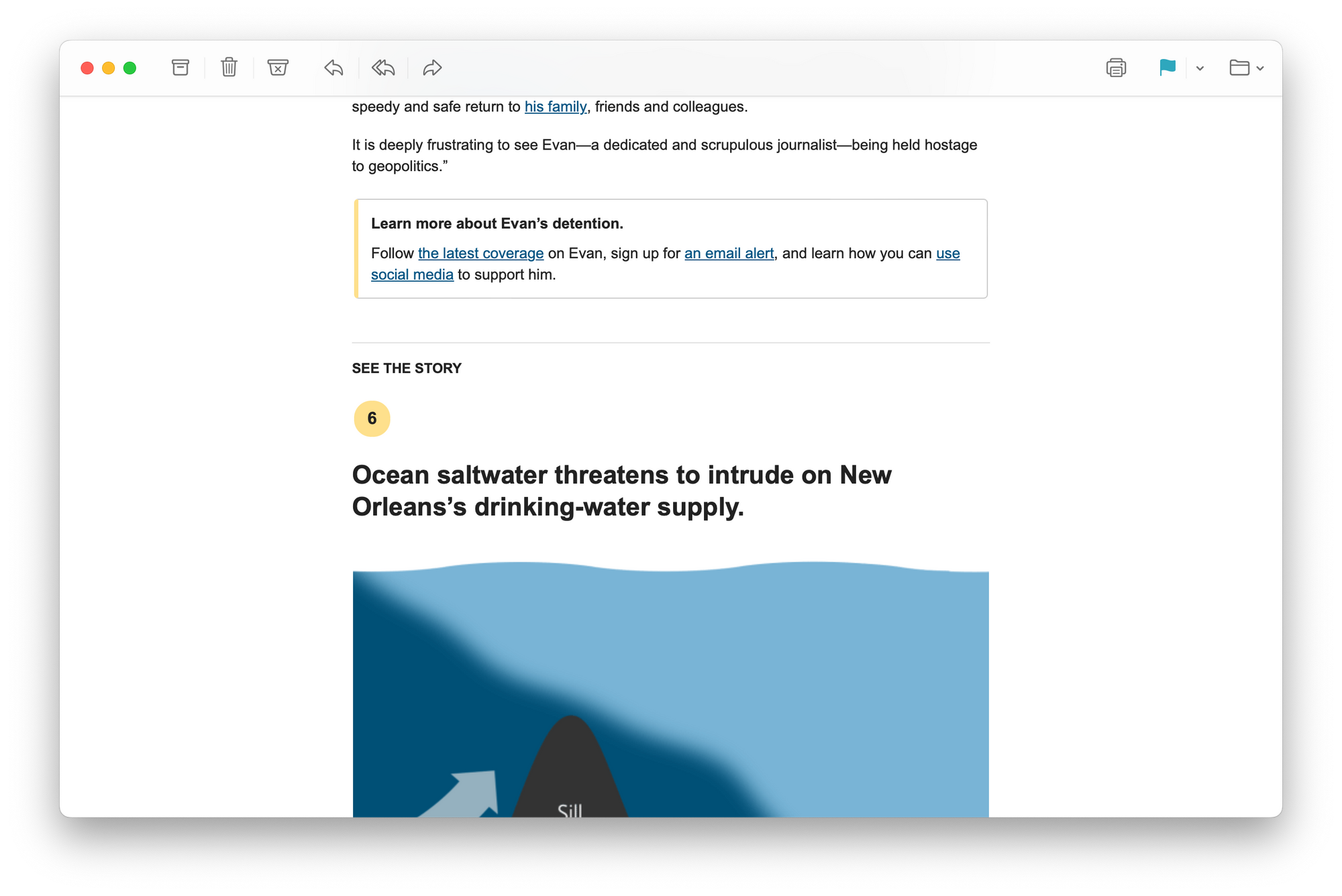The image appears to be a screenshot from either a website or an app. At the very top, there is a horizontal line with a variety of icons above it, arranged from left to right. These icons include:

1. A red circle
2. A yellow circle
3. A green circle
4. A filing box
5. A trash can
6. Another container with an "X" on it
7. A single arrow pointing left
8. Two superimposed arrows pointing left
9. A single arrow pointing right

On the top right corner above the line, there is an icon of a printer followed by a blue flag. There is a small vertical line separating these from a down arrow and a picture of a folder with another down arrow to its right. This section resembles a menu bar.

Below this, the background is white with some black text. The text reads, "speedy and safe return to his family," formatted in blue to indicate a hyperlink, followed by "Friends and colleagues." The next line states, "It is deeply frustrating to see Evan, a dedicated and scrupulous journalist, being held hostage to geopolitics."

Below this text, there is a box with a call-to-action including multiple hyperlinks:
1. "Learn more about Evan's detention"
2. "Follow the latest coverage on Evan"
3. "Sign up for an email alert"
4. "Learn how you can use social media to support him"

Further down, it says "see this story" with the number 6 inside a yellow box. Beneath that, there is a headline: "Ocean saltwater threatens to intrude on New Orleans drinking water supply." 

Under the headline, there is a partially visible image shaped somewhat like a flag, featuring light blue and darker blue colors along with a light blue arrow pointing northeast. Additionally, there is a hill depicted with some text on it, but the text is not legible.